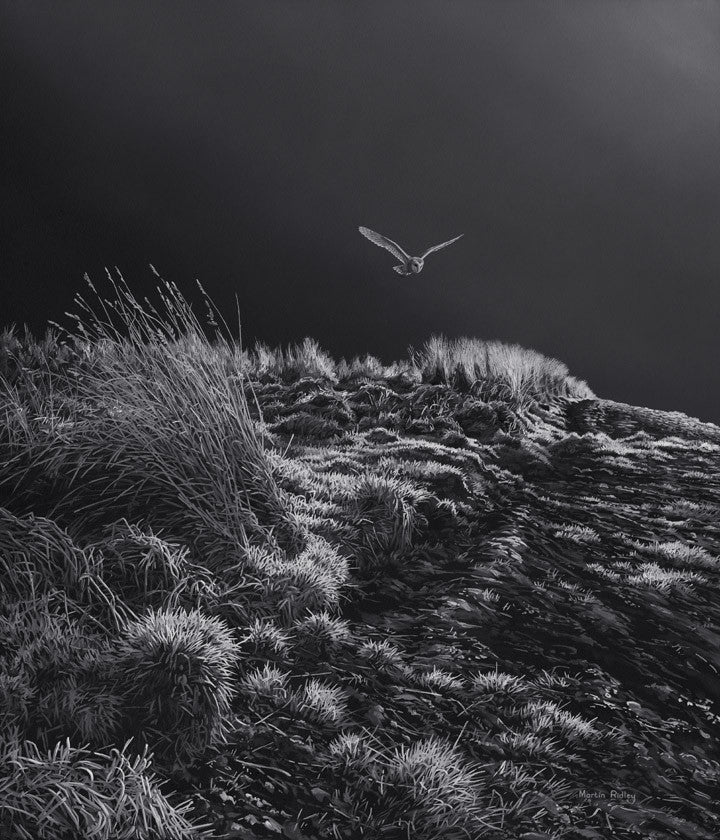This detailed black-and-white artwork, possibly a chalk drawing, captures a large owl in mid-flight over a grassy hill. The owl, outlined in white against a stark black sky, is positioned in the upper center of the image with its wings fully extended in a V-shape, soaring slightly upward and to the left. The owl's face is illuminated with a lighter shade, contrasting with its darker body, while its piercing eyes command attention. The hill below, constituting most of the foreground, is adorned with a mix of short and long grass, shrubs, and patches of dirt, evoking a wild, natural setting. A subtle light source, possibly hinting at moonlight, adds a sense of depth and atmosphere. The signature of the artist, Martin Ridley, is discreetly placed in the bottom right corner, marking this evocative piece.